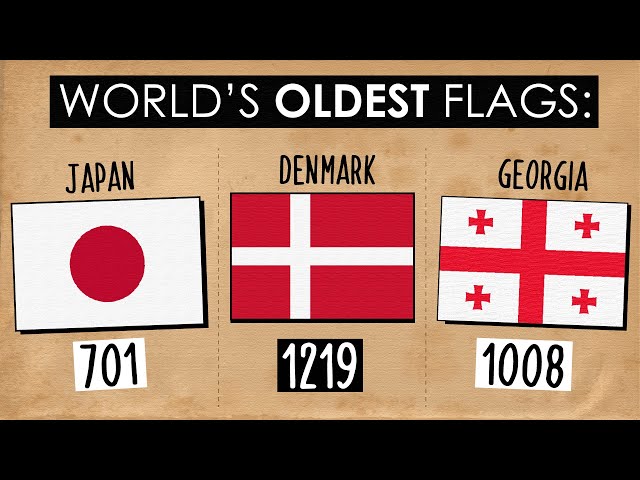The image is an infographic titled "World's Oldest Flags" set against a beige leather-looking background. It features three flags—Japan, Denmark, and Georgia—each accompanied by their respective ages: 701 years, 1219 years, and 1008 years, respectively. The top and bottom of the infographic have a black border, with the title in large white letters on a black rectangle at the top. The Japanese flag is depicted as a white rectangle with a red circle in the center, labeled "Japan" with "701" written in black text bordered in white. The Danish flag is shown as a red rectangle with an off-centered white cross to the left, labeled "Denmark" with "1219" written in white text on a black background. The Georgian flag features a white rectangle with a central red cross and additional red crosses in each quadrant, labeled "Georgia" with "1008" written in black text bordered in white. Each flag is distinctly red and white, and the infographic's layout highlights their unique designs and significant ages.